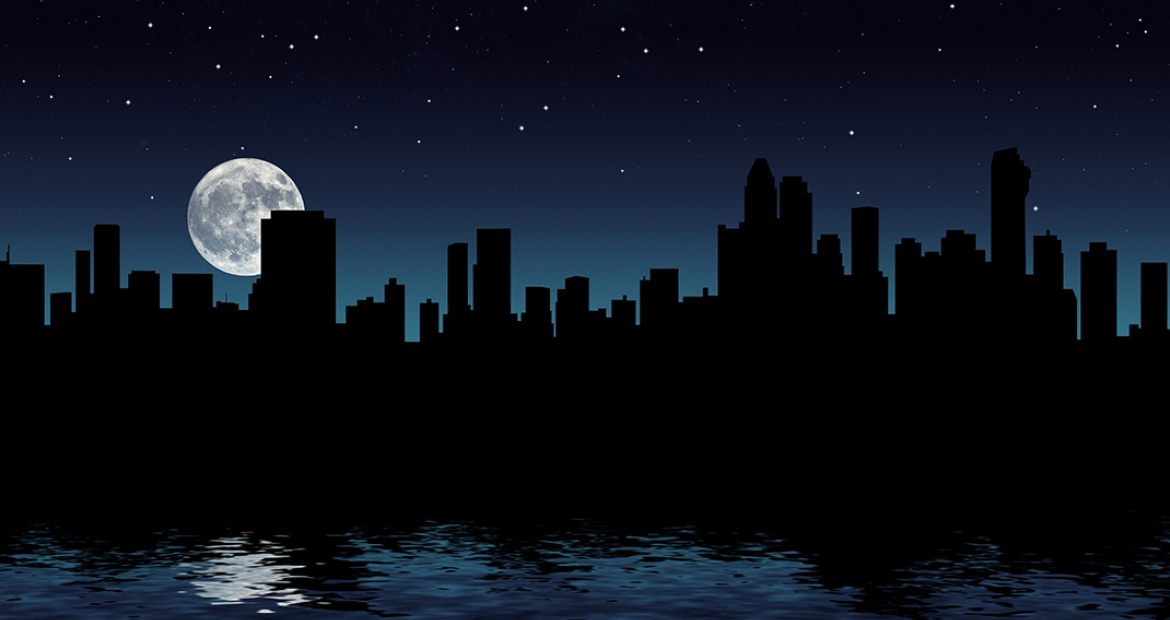This is a detailed illustration depicting a nighttime cityscape. The night sky, a gradient of dark to lighter blue, is adorned with numerous white stars, varying in brightness. Dominating the scene is a large, partially obscured moon, its mottled gray and white surface peeking from behind a towering skyscraper on the right. The skyline features an array of buildings of various heights, their silhouettes stark against the celestial backdrop. Beneath the buildings lies a tranquil body of water, capturing the reflection of both the illuminated skyline and the moon. The overall color palette is predominantly dark, with deep shades of blue and black, punctuated by the bright white of the stars and moon, contributing to the serene, nocturnal atmosphere.